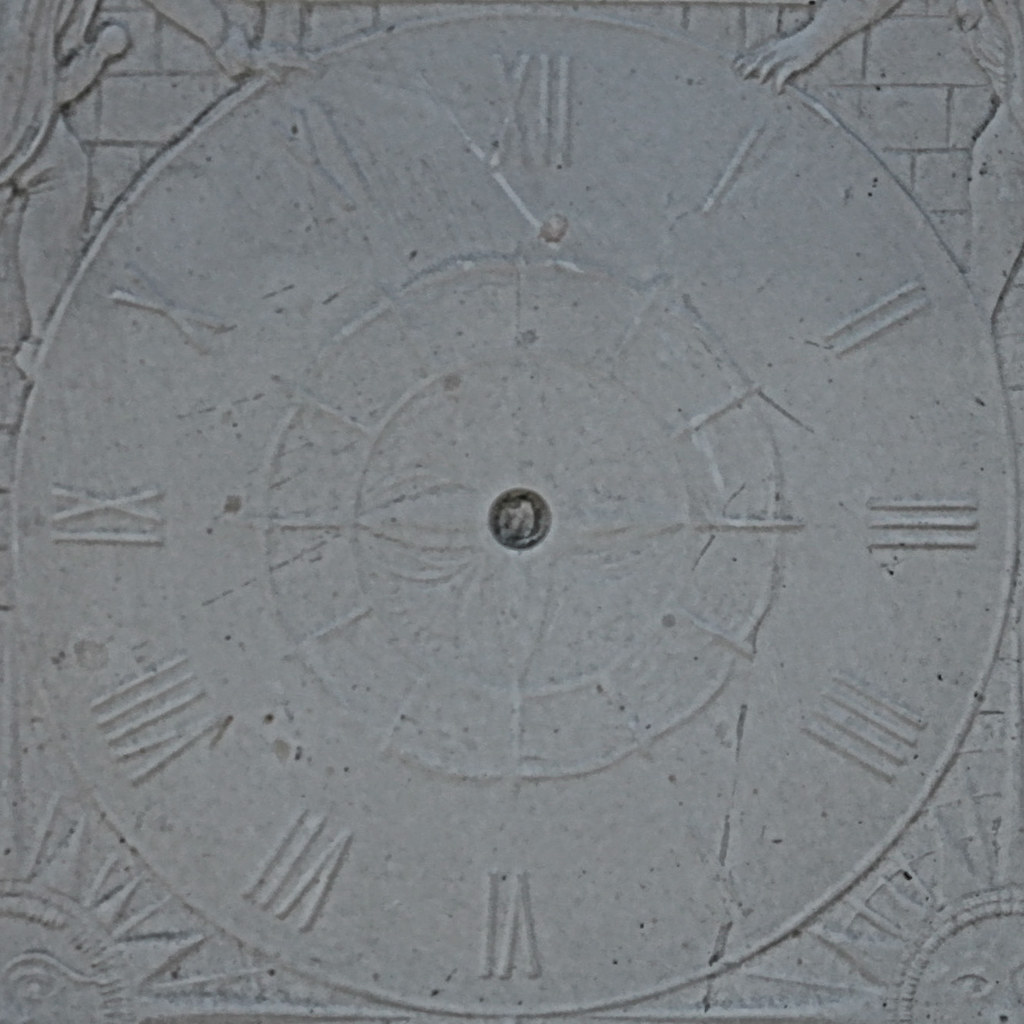The image depicts a highly detailed, yet aged and grainy close-up of a stone-carved clock face, whose surface is worn to the point that it obscures many of the finer details. The clock is circular, adorned with barely visible Roman numerals from 12 through 11, indicating its once functional nature. At the center, there is a faded black circle with indistinct gray markings, possibly where clock hands might have once been attached. Surrounding this central circle, one can observe a heavily eroded symbol that resembles a flower, though its exact design is unclear due to its faded state. 

On the lower left and right corners of the clock face, there are sun motifs featuring faces and radiating rays, almost like mini-suns carved into the stone. At the top left and right, part of human figures—arms, bodies, and legs—are visible, suggesting that these figures might be holding or reaching towards the clock. A brick wall texture forms the backdrop to these figures, adding another layer of intricate detail to this carved stone relic. Overall, the image captures an ancient, weathered artifact whose original purpose and design have been largely eroded by time.